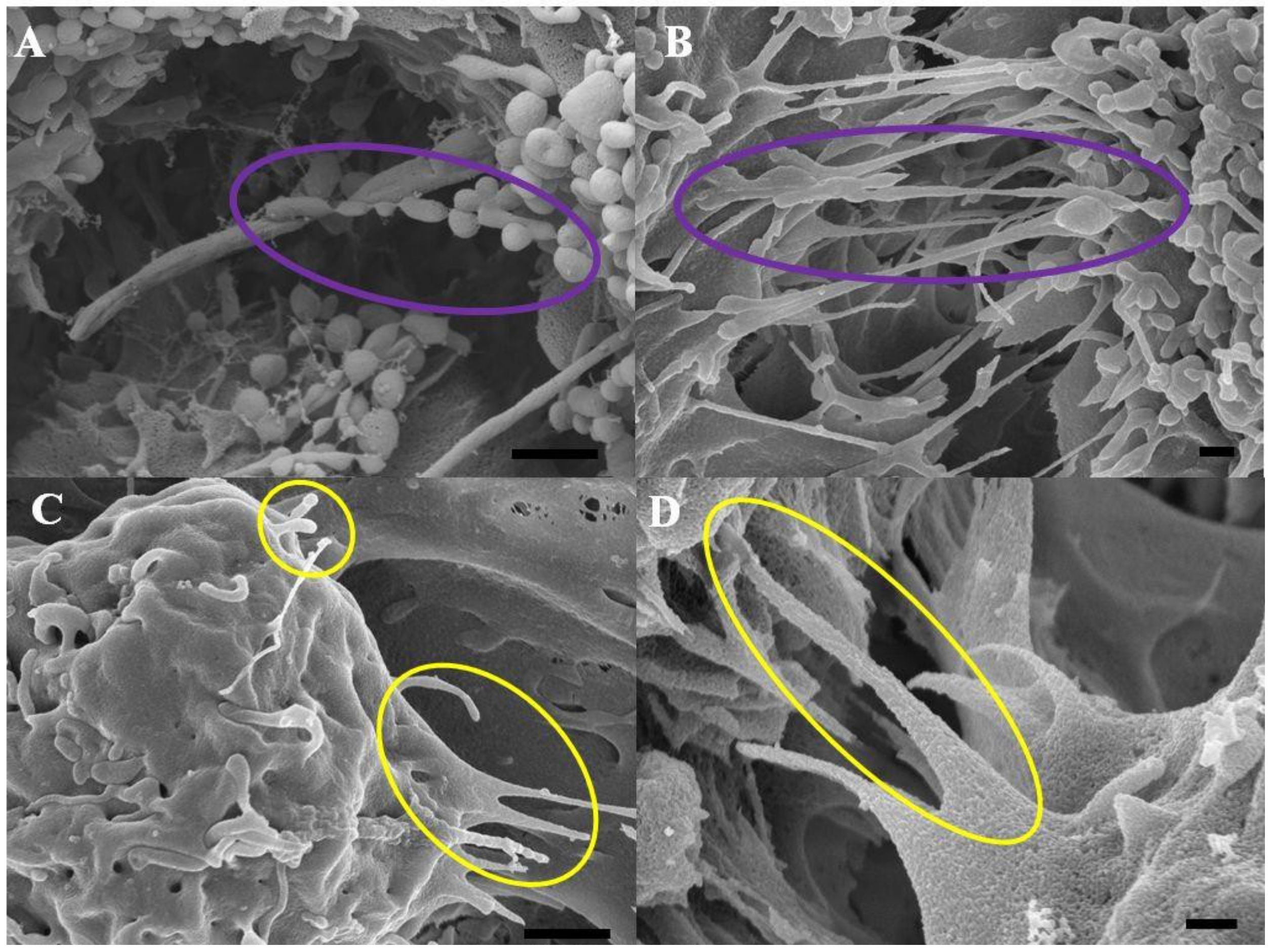This scientific black-and-white image is divided into four equal sections labeled A, B, C, and D, arranged in a two-by-two grid. Each section features a close-up microscopic view, likely of biological material, possibly bacteria or internal structures within an organism. In the top left corner (section A), a purple ring highlights a specific detail resembling a tunnel covered with round, white balls. The top right corner (section B) also has a purple ring around what looks like a chasm with white lines on either side. The bottom left corner (section C) features two yellow rings emphasizing particular spots on the bacteria-like structures. In the bottom right corner (section D), a solitary yellow ring identifies another point of interest. These highlighted sections suggest a specialized focus, likely for scientific or medical educational purposes.